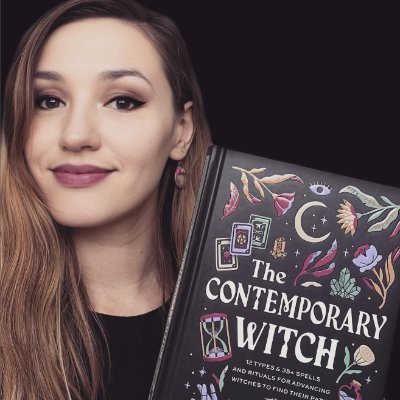In this perfectly square photograph, a young woman with long brown hair, brown eyes, and thick eyeliner, complemented by maroon lipstick, is positioned on the left-hand side. She gazes directly into the camera with a closed-mouth smile, the image cutting off just above her forehead and at her chest, revealing a black shirt. The background behind her is black, appearing slightly blurred at the edges as if Photoshopped. In the lower right-hand corner, she is holding a black book titled "The Contemporary Witch" in bold white text. The book is adorned with various colorful illustrations including a crescent moon surrounded by three stars, an eye shaped like a football, several flowers in hues of yellow, purple, and green, and three tarot cards. There is also an hourglass depicted among the vibrant images of yellows, reds, greens, and blues. The composition is devoid of any other people or text, focusing solely on the woman and the book she holds.